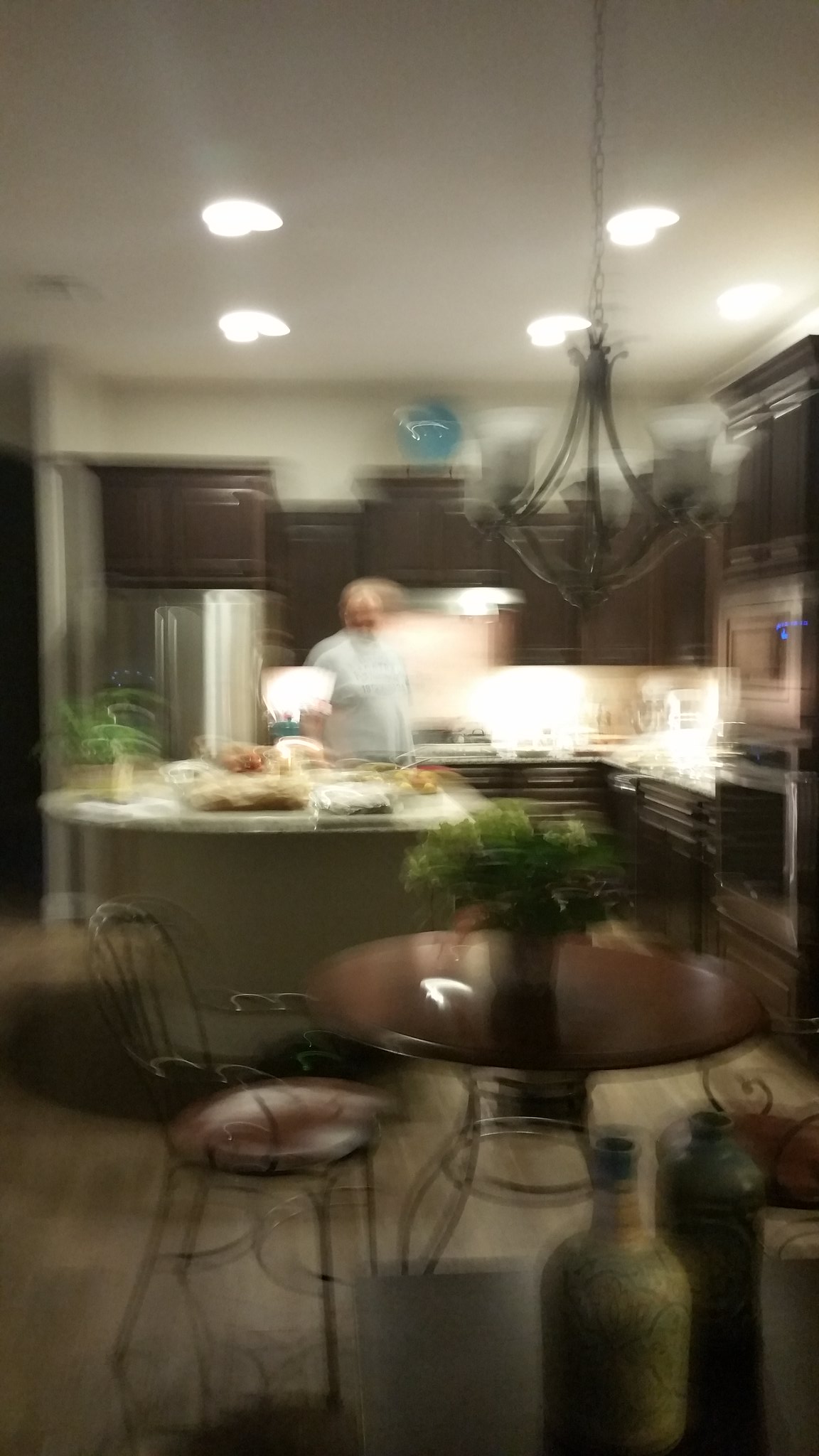This photograph, though extremely blurry and out of focus, captures a kitchen viewed from an adjoining dining room, suggesting that the picture was taken while in motion. The kitchen features dark brown cabinetry and various appliances including a silver refrigerator on the left, an oven with a microwave above it on the right, and a countertop island in the center. The island appears to have a beige and white base, and on top of it, there are some foods and a green plant. The ceiling, adorned with five round lights, also features a wrought iron ceiling fixture that might be a chandelier. 

In the foreground, there is a dark brown circular dining table with a bouquet of flowers and a couple of dark green and light green jugs placed on it. There are two chairs at the table, each with four legs. Standing in the kitchen is an older white male, appearing either bald or heavyset, wearing a light blue or gray shirt, though his face is indiscernible due to the blurriness of the image. The floor is wooden, and the countertops in the kitchen are white, adding contrast to the darker cabinetry and overall kitchen layout.